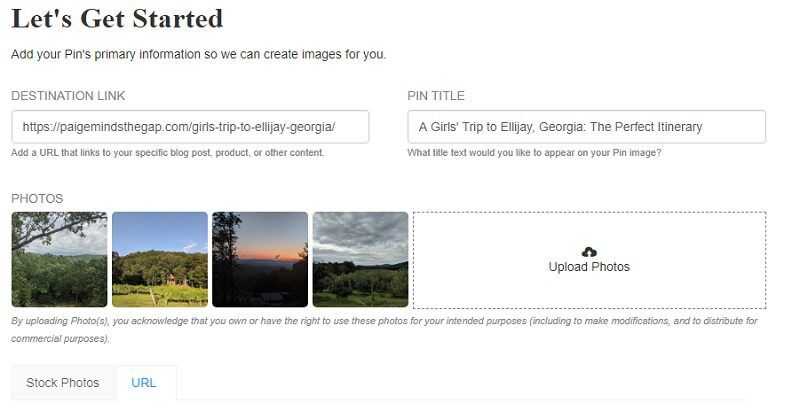The website interface depicted is a stock photo platform, guiding users through the process of creating customized images. At the top, a call-to-action banner declares "Let's Get Started" and instructs users to add their PINs (Primary Information Numbers) to facilitate image creation.

Below this, a dedicated field labeled "Destination Link" is visible, with a sample URL: "https://pagemindsthegap.com/girls-trip-to-lej-georgia/". A note beneath the field advises users to add a URL linking to specific content such as a blog post or product.

Adjacent to this, another text box titled "PIN Title" contains the entered text "A Girl's Trip to Lej, Georgia: The Perfect Itinerary," specifying the title that will appear on the resulting PIN image.

Further down, a section labeled "Photos" displays four thumbnail images: a treed mountain landscape, a field with a central house, a vibrant sunset with pink, yellow, and blue hues, and a stormy sky above an open field. Below these, an upload area is depicted with a cloud icon and arrow, set within a dashed border, indicating that users can drag and drop their photos. Text accompanying this area clarifies that by uploading, users confirm their ownership or right to use the images for modifications and commercial purposes.

Lastly, the interface includes two tabs: "Stock Photos" and "URL." The active tab, "URL," is highlighted in blue, while "Stock Photos" remains in black text, signifying that the user is currently in the URL section.